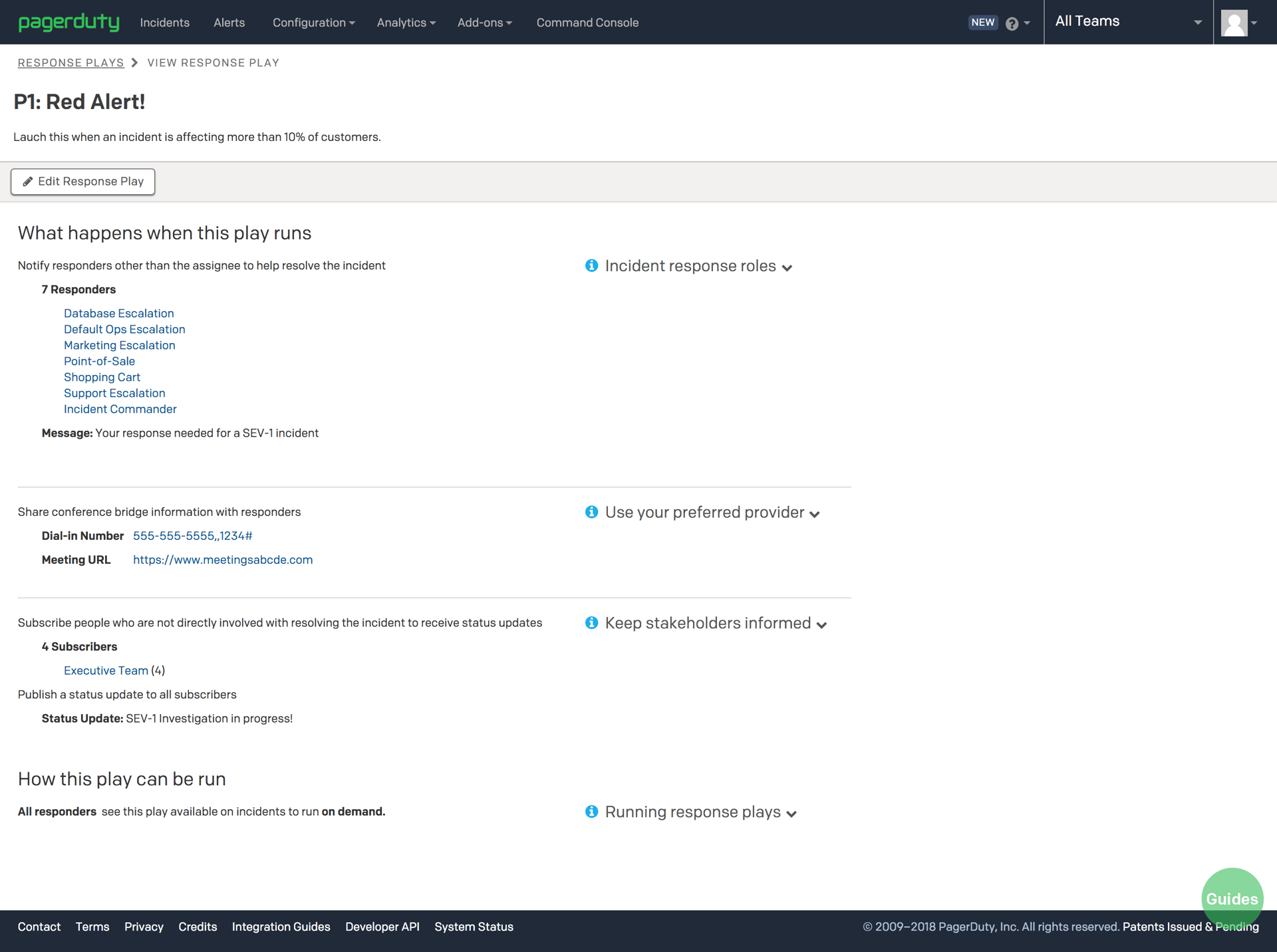**Detailed Descriptive Caption:**

The screenshot displays the interface of PagerDuty, a notable incident management platform, highlighted by its lowercase green logo at the top left. Adjacent to the logo in white text are various navigation options: "Incidents," "Alerts," "Configuration," "Analytics," "Add-ons," "Command Console," "New," and "All Teams." Below this navigation bar is a white section with black text detailing a specific incident response protocol. 

This section is titled "Response Plays," and delves into the "View Response Play" for a "P1 Red Alert," used when an incident affects over 10% of customers. There's an option to "Edit Response Play" and a question, "What happens when this play runs?" The play is designed to "Notify responders other than the assignee to help resolve the incident."

Under "Incident Response Roles," the document lists 7 key responder roles:
1. Database Escalation
2. Default Ops Escalation
3. Marketing Escalation
4. Point of Sale
5. Shopping Cart
6. Support Escalation
7. Incident Commander

The play additionally instructs responders to share conference bridge information via a dial-in number (555-555-5555) with pin 1234#, and a meeting URL (https://www.meetingsabode.com). There is an emphasis on using a preferred provider.

The instruction states to "Subscribe people who are not directly involved with resolving the incident to receive status updates," to "Keep stakeholders informed." Specifically listed subscribers include the Executive Team (4 members). It mandates the publication of a status update to all subscribers indicating that the "SEV-1 investigation is in progress."

The section titled "How this play can be run?" explains that "All responders see this play available on incidents to run on demand." Finally, the document talks about "Running Response Plays."

At the bottom is a black banner featuring several links: "Contact," "Terms," "Privacy," "Credits," "Integration Guides," "Developer API," "System Status," alongside a copyright notice for PagerDuty indicating the years 2009-2018, and mentioning "All Rights Reserved" with "Patents Issued and Pending."